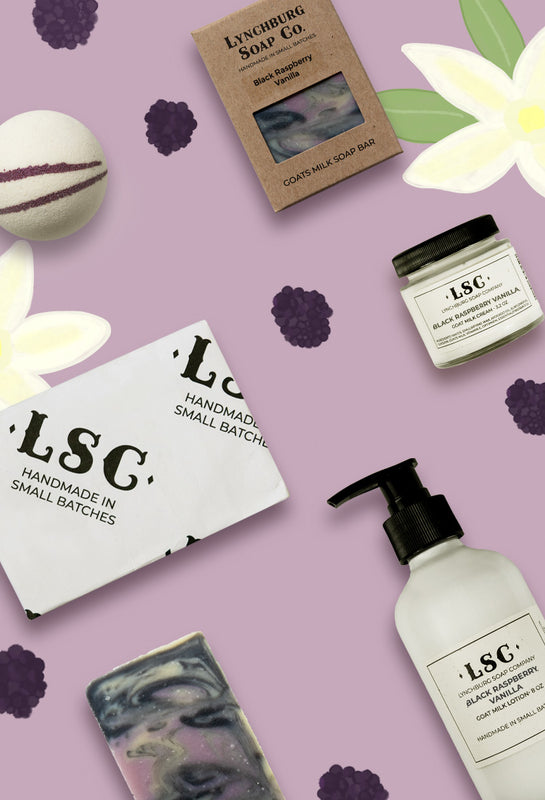The image displays a tall rectangle with a light purple background, showcasing a collection of products from the Lynchburg Soap Company, known for their black raspberry vanilla fragrance. On the bottom right corner, there's a clear bottle with a pump top, labeled "LSC Black Raspberry Vanilla Goat Milk Lotion, 8 ounces." Above it, to the left, is a white square, slightly tilted, featuring "LSC" in black text, along with "handmade in small batches." In the upper right corner, there is a delicate white flower with a yellow center and green leaves, accompanied by a brown book with "Lynchburg Soap Company" written on it. Nearby, a glass container with a black top and a white label also bears the "LSC" logo. On the far left side, a white circular ball with purple lines complements the background, which is adorned with dark purple berries. The arrangement of these objects gives the image a clean, fresh vibe, enhanced by the lavender hue of the background and the harmonious scattering of flowers and berries.